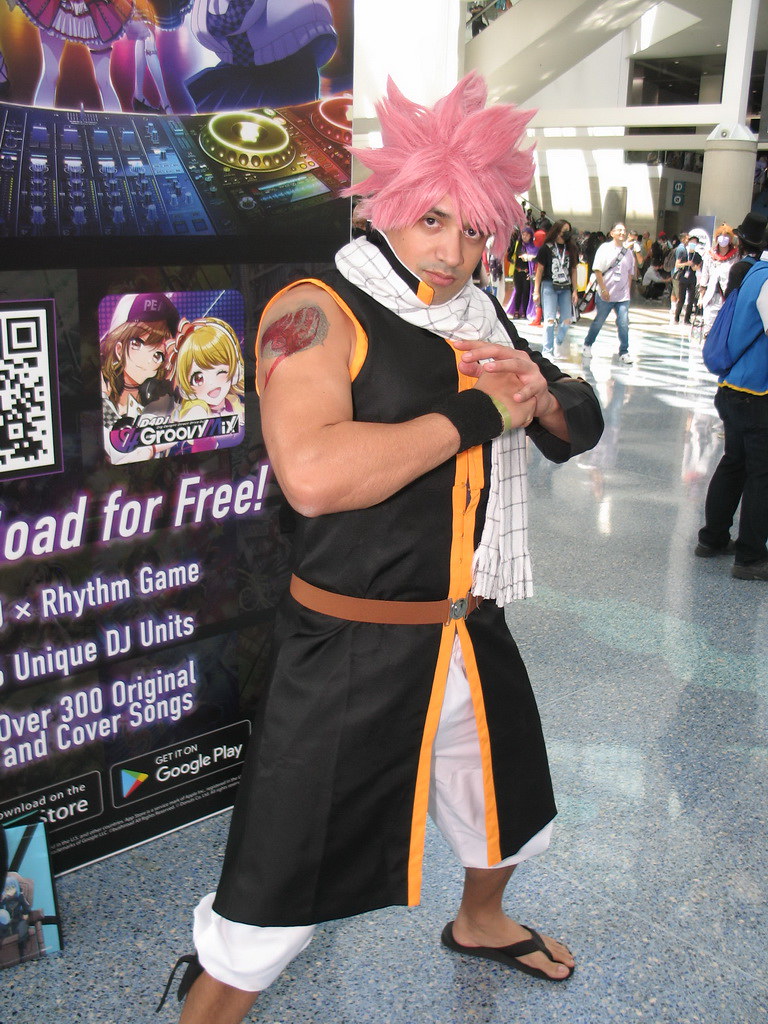In the bustling atmosphere of a convention center, a young man in his early 20s is captured in a striking portrait. He stands confidently in an attack pose, hands crossed on his chest, embodying a character from an anime. He wears a light pink spiked wig and a black kimono-like robe with orange trim, held together by a brown belt with yellow piping. His outfit is completed with white pants and traditional sandals. A white scarf drapes around his neck, and a prominent tattoo adorns his upper right arm. Behind him, a vibrant vertical poster featuring manga-style animated characters promotes a rhythm game with text that reads, "For free. Rhythm game. Unique DJ units. Over 300 original and cover songs. Download on the Apple Store and get it on Google Play." The scene is set in an indoor courtyard with light, hard floors, white pillars, and walls, filled with other convention-goers—some dressed in everyday attire and others in elaborate costumes. This detailed photograph captures the essence of a dynamic convention environment, blending elements of fantasy and reality.